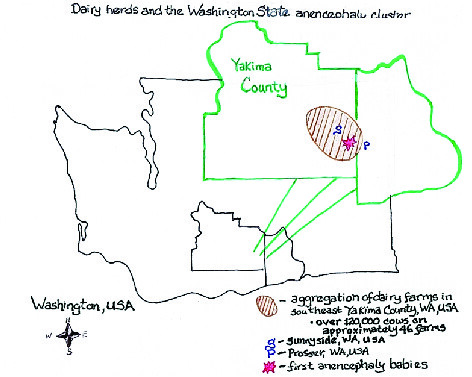This image is a detailed hand-drawn map focusing on dairy herds in Washington State. At the top, it prominently reads "Dairy Herds in Washington State" in black letters. The map features a black-and-white layout with some color accents. There is a highlighted blow-up section of Yakima County, outlined in green, containing a pink, diagonally-striped, egg-shaped area with a small red star at the bottom. In this section, there are the letters "S" and "P" in blue. Below the main map, on the left, the text "Washington, USA" is accompanied by a small compass logo. To the right, a key details the map's notations, explaining various symbols. This includes a notation about an aggregation of dairy farms in Southeast Yakima County, indicating over 20 farms. Additional descriptions involve specific locations marked "G" for Gunnyside and "P" for Prosser, Washington, USA.